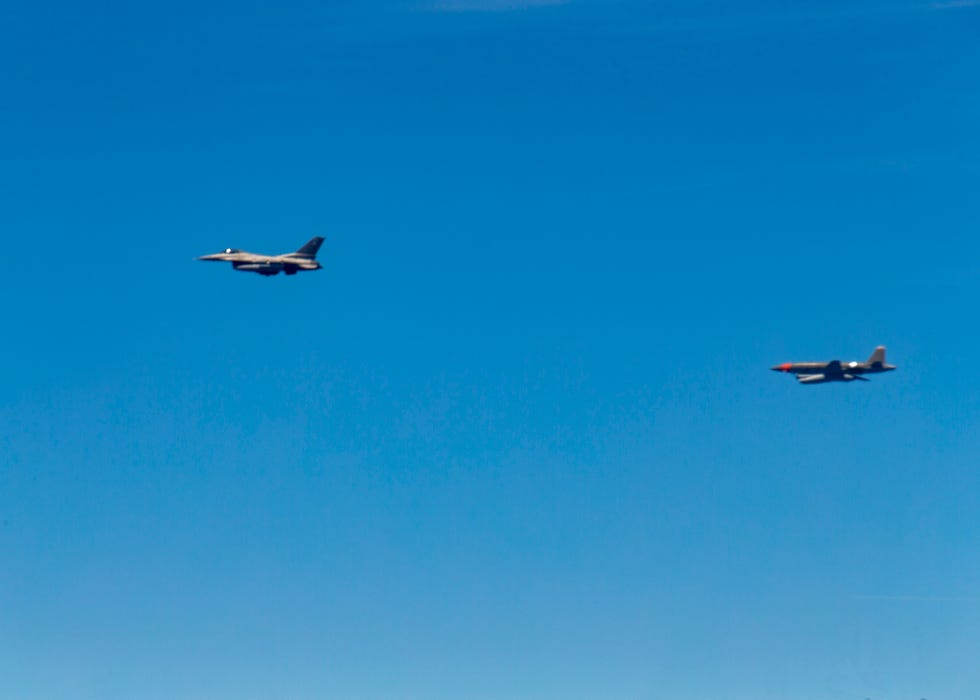This slightly blurry, large square photograph captures two fighter jets flying against a mostly clear blue sky. Both jets are distinctly positioned: the left jet, situated in the upper middle quadrant, has a gray body with a dark gray or blue tail fin and appears to be reflecting some light off its black canopy. It's possibly an American model, like an F-15 or F-16, seen from the side as it flies towards the left. The other jet, lower and more towards the right, also has a gray body but is characterized by an orange-tipped nose and a red cockpit area. Both jets are flying in the same direction through a sky adorned with faint, feathery lines of white clouds scattered subtly near the top and middle parts of the photo. The overall composition highlights the jets against the nearly pristine, light blue sky.